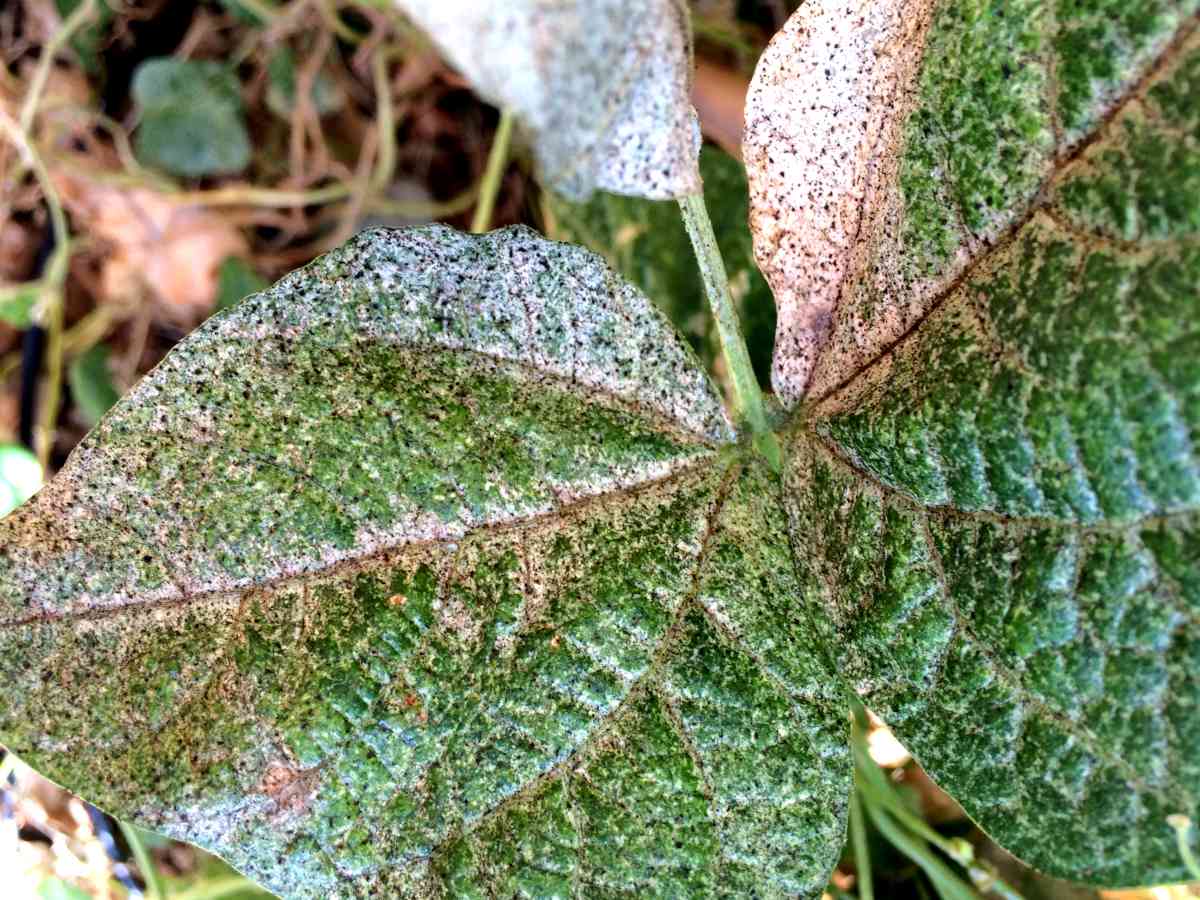This close-up, full-color photograph captures the intricate details of a partially withered leaf from a plant with a distinctive five-leaf cluster arrangement. The focal point of the image is one of these star-shaped clusters, where four leaves overlap closely, while the fifth leaf, either bending backwards or on a longer stem, appears slightly separated from the rest. The leaf surfaces exhibit a rough texture with a network of veins and indentations highlighted by high contrast lighting. The leaves predominantly show green coloration interspersed with speckles of black and brown spots, suggesting a degree of aging or disease. Some veins appear brownish, while white speckling is noticeable near the stem and around the veins. The background includes other green leaves, stems, weeds, and remnants of dead leaves on the ground, adding depth to the image captured from above.